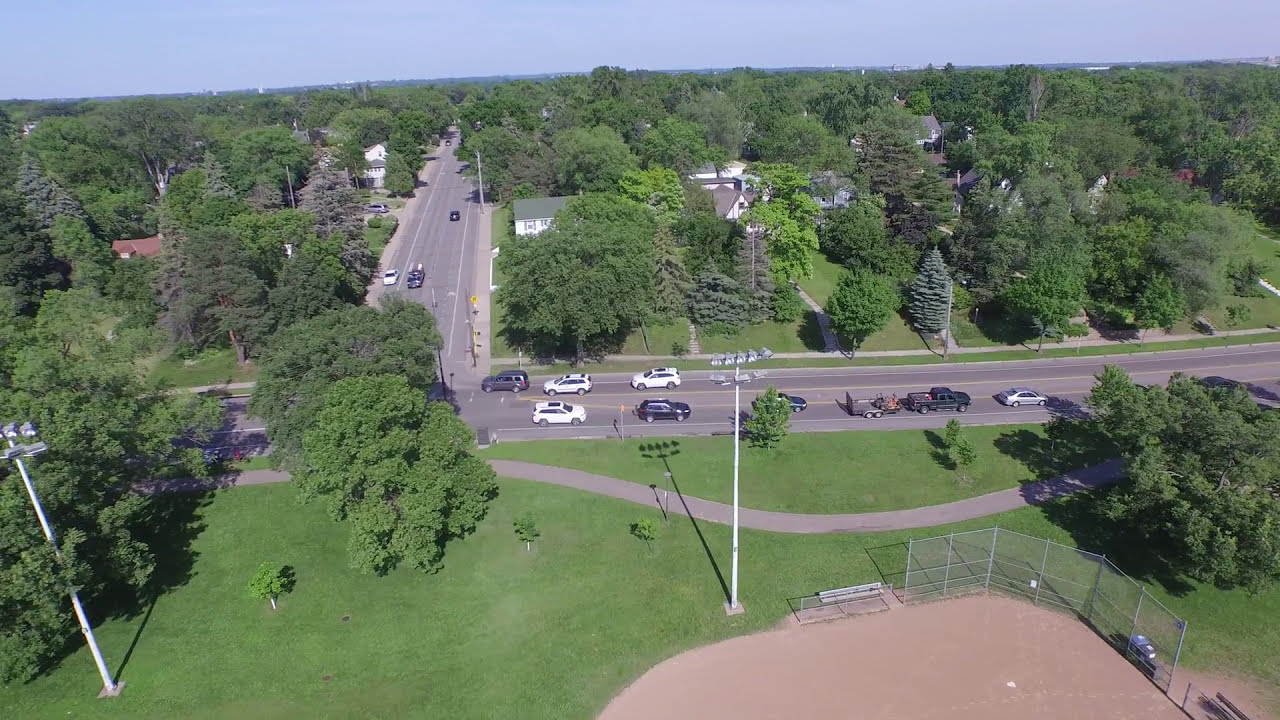This aerial photograph captures a tranquil neighborhood nestled within an abundant spread of green foliage, characterized by a plethora of trees that dominate the landscape. The homes are scattered amidst this verdant setting, each situated on individual grassy plots that blend seamlessly with the wooded surroundings. A winding road weaves through the scene, forming a T-shape and hosting a mixture of parked and moving vehicles, with a count of roughly 15 cars in total.

In the foreground, there is a baseball field surrounded by a silver metal fence, likely serving as a practice field given the lack of large outer fencing typical of professional fields. The field is equipped with tall stadium lights, ready to illuminate it during night games, though the scene is captured in broad daylight under a clear, sunny sky.

Completing the pastoral charm, a winding sidewalk encircles the field, enhancing the communal feel of the area. The high vantage point of the photo offers a comprehensive, almost bird's-eye-like view, ensuring a sweeping look at this serene and picturesque town scene.